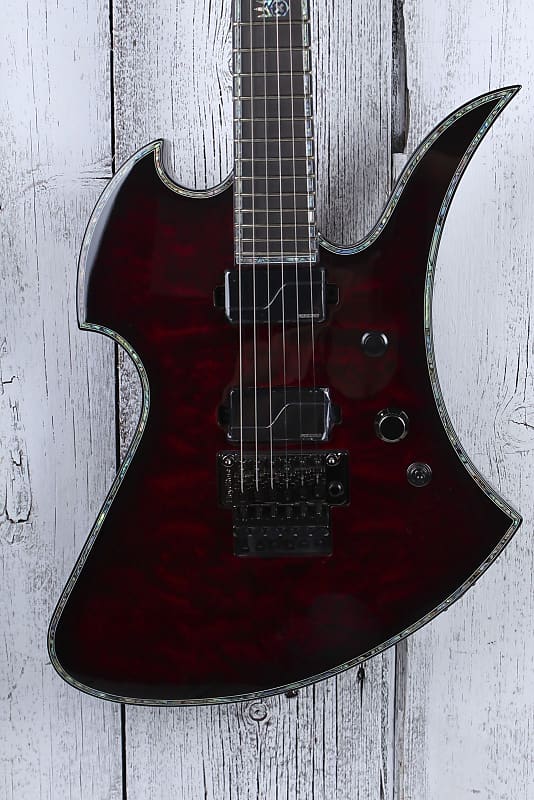This is a striking stock photograph of a uniquely designed electric guitar set against a worn white wooden plank background. The guitar features an angular and sharp silhouette, evocative of a fireball, with uneven, flame-like edges. Made from deep, dark cherry mahogany wood, the body showcases a rich variance of colors and a glazed finish, complemented by a silver lining that extends up the neck. The guitar has six strings and a black fretboard. There are three control knobs on the right side: a switch on the bottom and two knobs above it. The guitar is notably without a strap and appears to be hung against the white, slightly worn planks, which serve as a contrasting backdrop. The bottom half of the neck and the area where the strings are attached feature black detailing, adding further depth to the instrument's striking design.